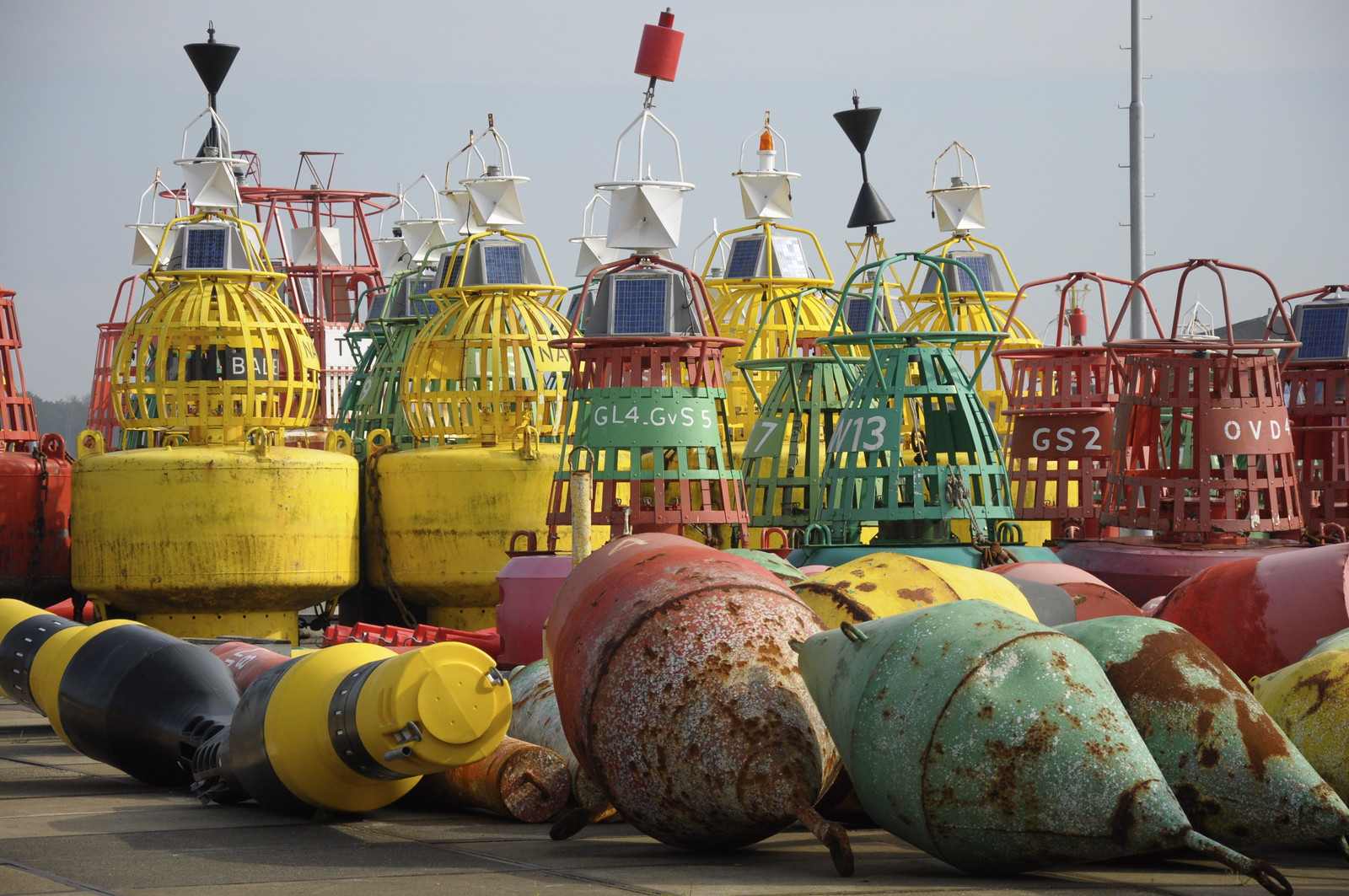The photograph depicts an assortment of buoys stored on a pier, featuring a variety of types, sizes, shapes, and colors. Prominently displayed in the foreground are buoys with a slightly rusty appearance, some mimicking the shape of Christmas lights. Colored in hues of green, red, black, and yellow, these buoys lie on their sides, showcasing signs of wear and age. Of particular note are a few modern synthetic buoys, characterized by their high-tech design, with striking black and yellow bottoms. The larger buoys in the background display solid bottoms with metal wire tops and protruding pieces, painted in shades of yellow, green, or red. Many are topped with white and adorned with different colored shapes. Several buoys are equipped with solar panels, presumably to power warning devices or lights, and feature metal bands inscribed with numbers and letters like GL4, GVS5, GS2, and OVD. Some buoys also have red blinking lights and cone-shaped horns, likely for use in foggy conditions. The entire scene is set against a cloudy sky with trees visible in the background, emphasizing the buoys' readiness for deployment in navigational settings.